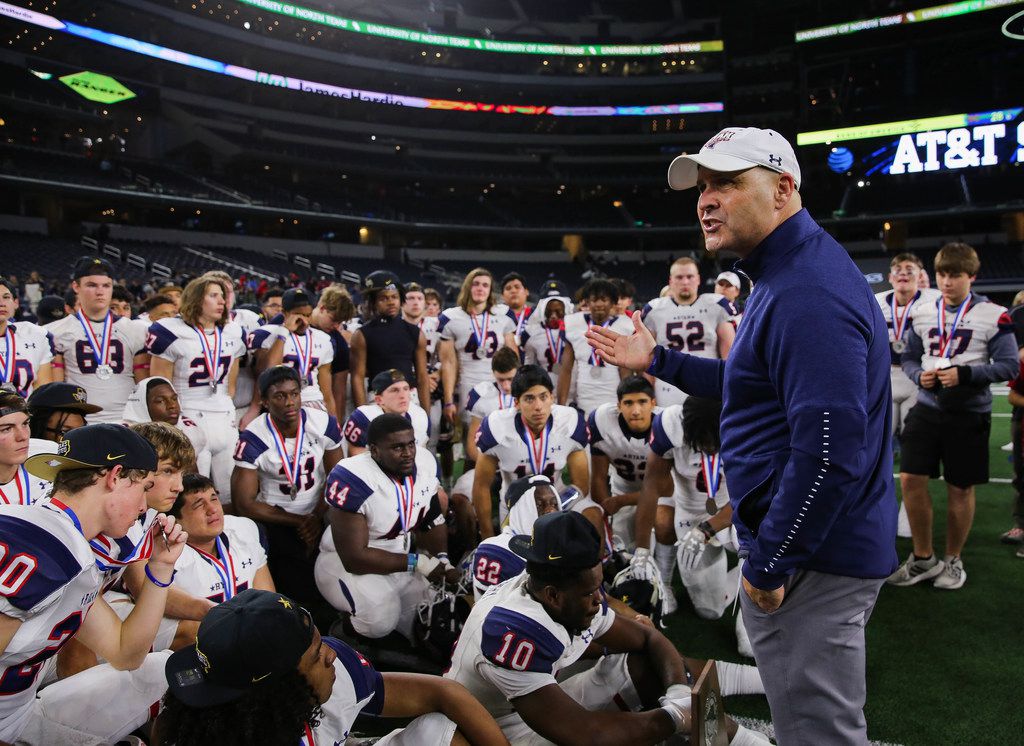In this image, a head coach, sporting a white hat and a blue long-sleeve jacket with a collar, addresses a group of kneeling football players at AT&T Stadium, home of the Dallas Cowboys. The players, seemingly young, possibly from a high school or college team, wear white uniforms with blue sleeves highlighted by white numbers outlined in red. Each player also has a medal around their neck, suggesting they have won a tournament. The background features the stadium's signature lights and ticker tape displays, enhancing the celebratory atmosphere as the coach gives an inspirational pep talk. The players' uniforms prominently feature blue letters with a red border, and the stadium displays, including the "AT&T Stadium" and "Ranger," can be seen in the distance, adding to the grandeur of the moment.